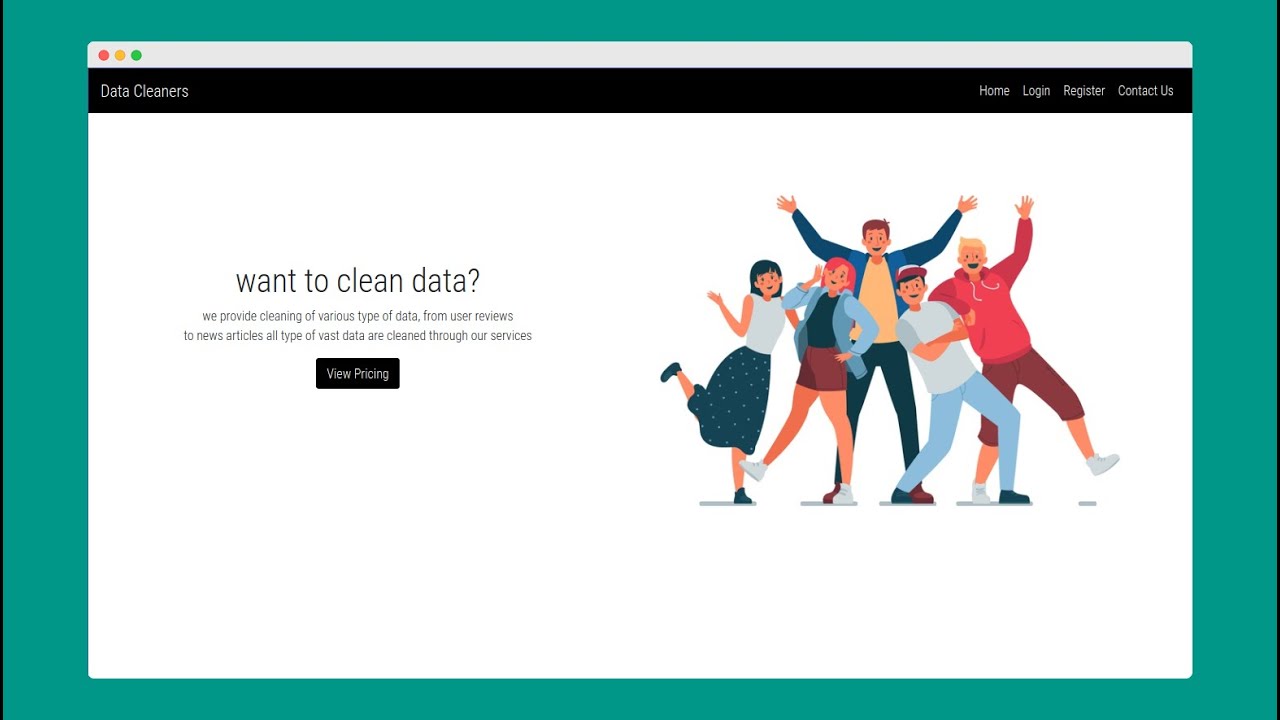This screenshot, captured from a Macintosh computer, is identified by the distinctive tan background and the light gray bezel framing the display. At the top of the screen, the familiar Mac control buttons—a red circle, an orange circle, and a green circle—are positioned, replacing the traditional minimize line, maximize square, and close "X" icons found on other operating systems.

Beneath this bezel, a black rectangle hosts the text "Delta Cleaners" in white on the left-hand side, and several clickable buttons on the right-hand side: "Home," "Login," "Register," and "Contact Us." Below, a white section prominently displays the bold heading "Want to Clean Data?" followed by a description in regular black text: "We provide cleaning of various types of data, from user reviews to news articles, all types of vast data and cleaned through our services." There’s also a "View Pricing" button contained within a black rectangle with white text.

On the right side of the screenshot, a group of cartoonish characters is featured. The first character is a light-skinned female with short blue hair, wearing a gray shirt and a blue skirt or dress adorned with white stars, complemented by blue shoes. Next to her is a character with reddish skin and red hair, dressed in a two-tone blue jacket over a dark blue shirt, a maroon skirt, and white shoes. Another character, a Caucasian male with short brown hair and outstretched arms, is shown in a dark blue long-sleeved shirt over a lighter blue vest, with a cream-colored undershirt, black pants, and brown shoes. Leaning towards him from the right is an olive-skinned male, donning a gray shirt with darker gray sleeves, a white and red hat, black shoes, and crossed arms. The final character, also light-skinned, smiles and raises his hands while wearing a red sweatshirt with dark red sleeves and maroon shorts down to his kneecaps, along with white shoes. Each character casts a shadow at their feet, adding depth to their depiction.